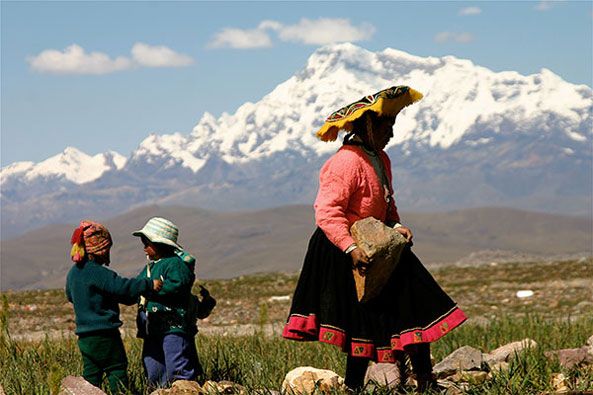This outdoor photo captures a native Latin American woman and her two young children as they work and play in a grassy field surrounded by stones. The woman, possibly of Inca heritage and dressed in traditional attire, is seen holding a large gray stone while constructing a short stone wall. She wears a black dress with red border edging, a thick wool-like top, and a sun hat adorned with black, red, white, and green designs, with a gold fringe. To her left, two children are playing; one is dressed in a colorful hat, a dark green long-sleeved shirt, and forest green pants, while the other wears a white and blue striped hat with a matching long-sleeved shirt and blue pants. Another child is faintly visible in the background with a finger extended towards their face. The scene is set against a picturesque backdrop featuring a mountain landscape, with tall, snow-capped peaks, green hills, and a clear blue sky scattered with white clouds.